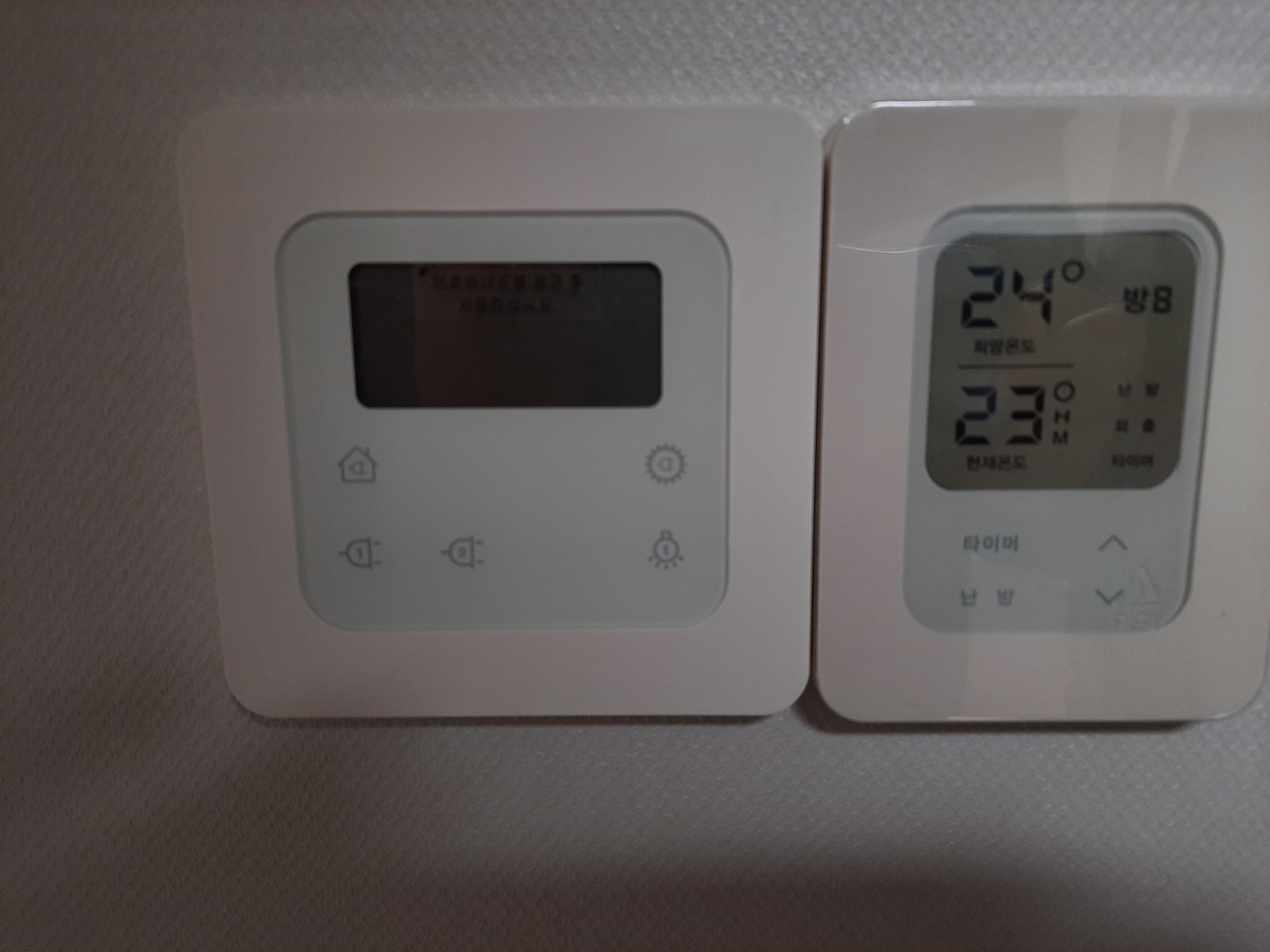This photograph, taken in a low-light indoor setting with overhead lighting from above and slightly behind the photographer, captures the shadow of a person casting against a textured wall, holding a phone with both hands. Details in the shadow suggest that the middle, ring, and pinky fingers of the left hand are raised as they grip the phone.

The image prominently features two digital display units mounted into the wall, which is adorned with wallpaper that showcases a fine diamond-shaped texture. The unit on the left has a broad, white plastic border encompassing a touch-screen display, which is inactive and completely dark. Surrounding the dark screen, within the pale blue area, are several buttons depicting symbols that are hard to discern but include icons resembling plugs, an on/off switch, and a light symbol.

To the right, there is a narrower, more rectangular display unit with a similar white border. This screen is illuminated with a pale grey background and features black digital writing. It reads "24 degrees" at the top and "23 degrees" below that, followed by abbreviations "H" and "M." Below these numbers, some text is present but not clearly legible. The bottom of the screen displays a series of indistinct symbols alongside up and down arrow controls.

This detailed composition meticulously captures the interaction between low ambient lighting, the reflective surface of the screens, and the tactile design elements of the units.